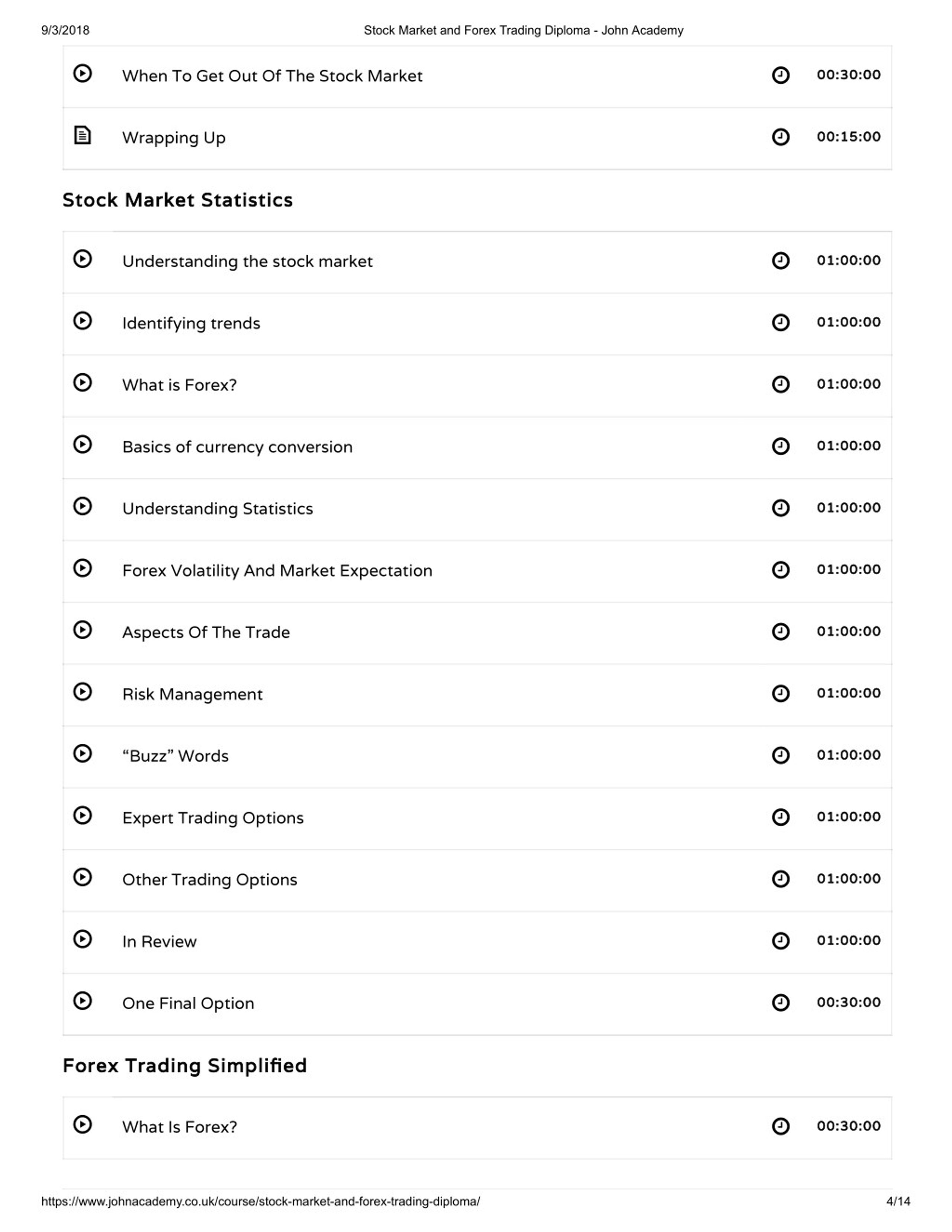A detailed timetable or syllabus displayed on a white background with black text outlines a comprehensive series of videos or classes focused on finance topics ranging from the stock market to foreign exchange (Forex). On the right side of each listed item, durations are provided, with some sessions lasting one hour and others 30 minutes. The content appears to cover an extensive curriculum, starting with "Understanding the Stock Market" and including segments on "Identifying Trends," "What is Forex?," "Basics of Currency Conversion," "Understanding Statistics," "Forex Volatility," "Aspects of the Trade," "Risk Management," "Buzzwords," and "Expert Trading Options." Towards the end, there's a mention of various trading alternatives and an interview segment, concluding with a final option. Below this main list, an additional standalone class titled "Forex Trading Simplified" is highlighted, indicating a dedicated focus on foreign exchange education.